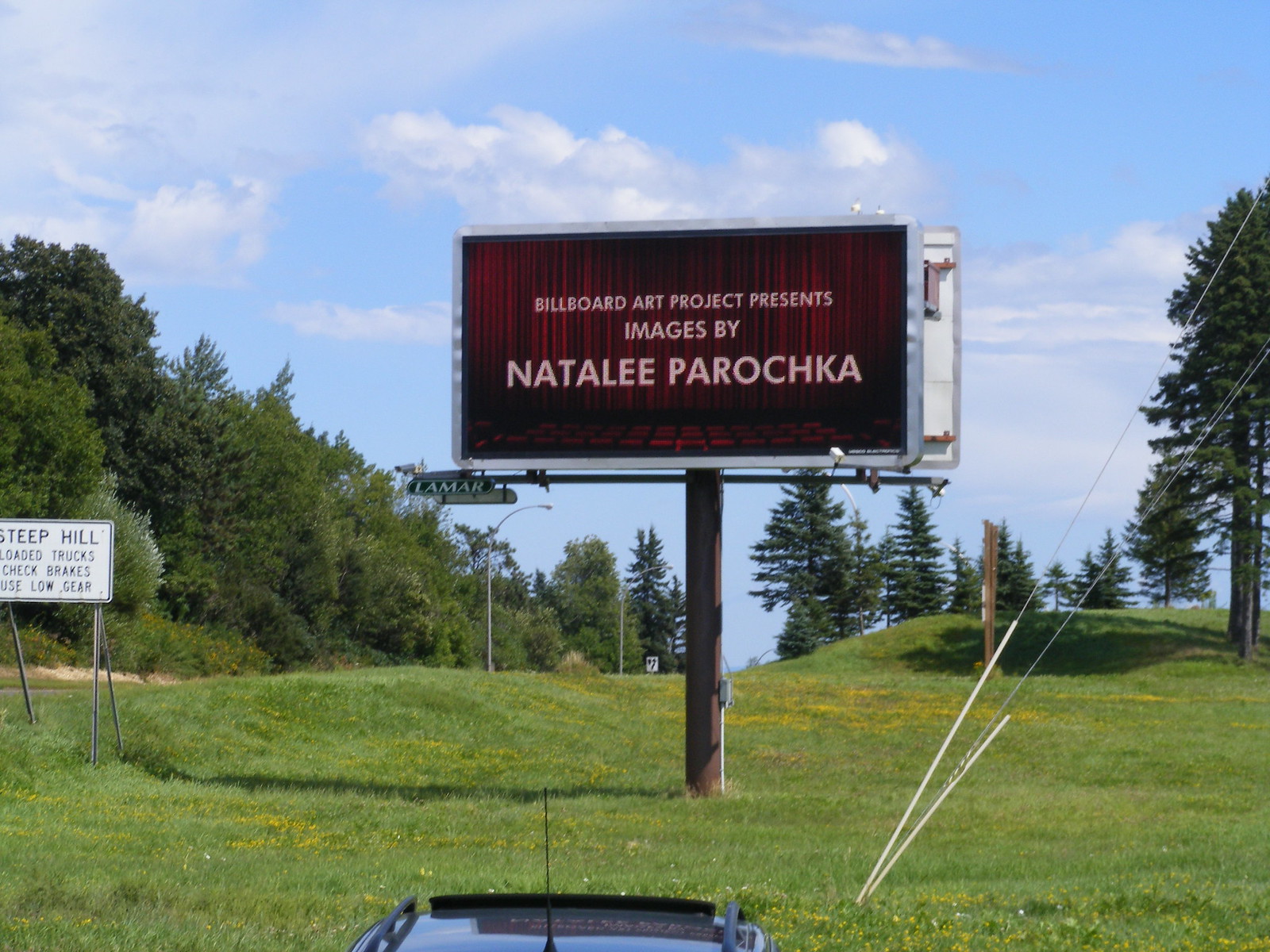This photograph captures a prominently displayed billboard situated in the center of the image. The billboard, mounted on a sturdy wooden pole, stands in the middle of a grassy field. The billboard reads in large, all-caps white lettering against a dark reddish-black background: "BILLBOARD ART PROJECT PRESENTS IMAGES BY NATALEE PAROCHKA." The largest text on the billboard spells out the artist's name, "NATALEE PAROCHKA," ensuring clarity with the distinctive spelling "N-A-T-A-L-E-E P-A-R-O-C-H-K-A."

In the foreground, the rear of a car is partially visible, adding a sense of scale and everyday context to the scene. The background features a row of lush green trees, complementing the natural setting. Above, a vibrant blue sky is speckled with numerous white clouds, casting a gentle light over the entire scene. On the left side of the image, another white sign with black lettering reads, "STEEP HILL LOADED TRUCKS CHECK BRAKES USE LOW GEAR," though it remains a secondary element to the primary focus on the billboard.